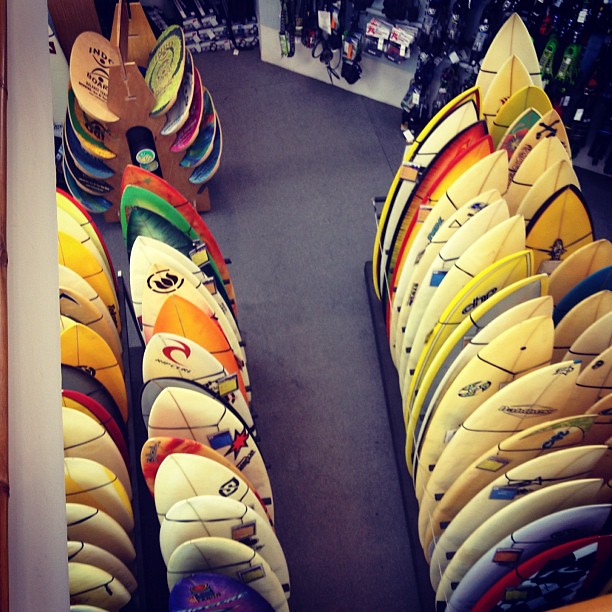The image is a color photograph taken from an elevated vantage point, likely the second floor or ceiling, looking down into the main floor of a surf shop. The square photograph captures an organized arrangement of surfboards and boogie boards within the store. Most surfboards are vertically stored in standing racks. Two main surfboard racks are visible: one in the lower left corner and another along the right side, each holding approximately two dozen surfboards in two side-by-side rows. The surfboards predominantly feature white backgrounds with decorative decals, though some are red, orange, green, yellow, black-rimmed, or solid blue and green—showing a vivid array of colors.

Central to the image is an A-frame wooden rack specifically designed to hold boogie boards. These boards, flatter and rounded compared to surfboards, are slotted into notches in the structure. The floor of the shop is covered in gray tiles or carpet squares, adding to the tidy appearance of the store. In the background, a wall rack displays various surfing accessories, including harnesses and leashes that probably connect surfers to their boards. The shop's meticulous layout and colorful equipment create a visually engaging scene for any surf enthusiast.